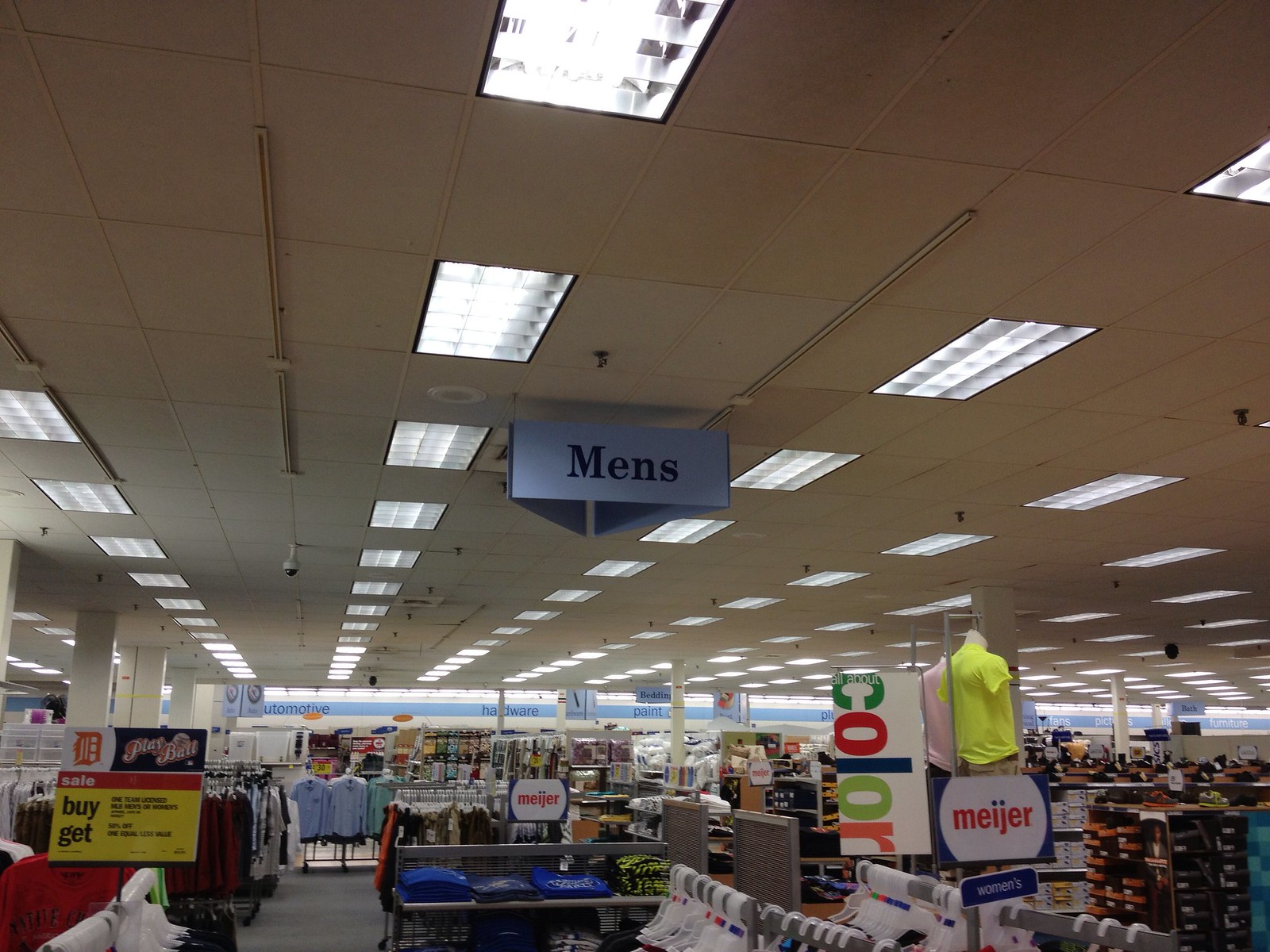This detailed image captures the interior of a department store, specifically a clothing section. The white-tiled ceiling is adorned with multiple rectangular fluorescent lights, water sprinklers, and security cameras. A prominent blue sign with black text hangs from the ceiling, indicating the "Men's" section. Beneath this sign, the store's layout includes aisles flanked by racks of clothes, with shirts displayed both on hangers and neatly folded on shelves. In the foreground to the right, stacks of shoe boxes are visible. There are colorful signage elements too; a rectangular white sign marked "color" in vertically arranged letters, each in a different color, and a nearby "Meijer" sign. The background features a white wall with a blue stripe and sections labeled for other departments, adding depth to the scene.